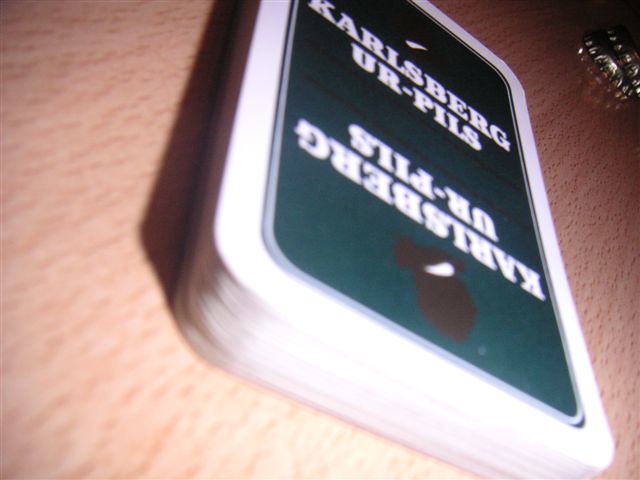This photograph, although somewhat blurry, features a light brown table with darker brown accents and a pattern of small lines and dots across its surface. In the upper right corner, the image darkens considerably, almost appearing black. 

Prominently displayed are two beer caps, which are silver and black with a shiny reflective surface. 

In the center of the image lies a deck of cards, positioned face down. To the left of the deck, a shadow can be seen. The cards have a white border with a dark blue center and a black circular emblem. The inscriptions "KARLSBERG" and "URPILS" are repeated twice on the deck.